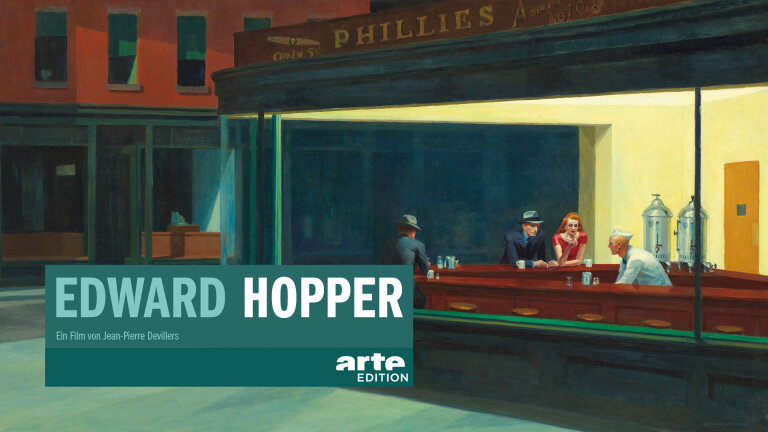This highly detailed scene depicts a stylized painting of a vintage diner with a distinct 1940s or 1950s aesthetic. To the right, there is a building featuring a glass wall, resembling a city cafe named "Fillies." A triangular-shaped bar occupies the center, surrounded by bar stools in a teal greenish-blue color, complementing the sidewalk's light green hue. The top portion of the building's exterior is red while the bottom is green. 

At this bar, a man and a woman sit closely together, engaged in conversation. The woman, with striking bright red hair, dons a fancy red dress. Beside her, the man is dressed in a navy blue business suit and a gray hat. Another man, distinguished by his gray suit and hat, sits further down the bar with his back to the window, facing the viewer. Separate from the couple, he appears isolated as no one is seated near him. 

In the center of the bar, the bartender, clad in a white shirt and a traditional white folded hat reminiscent of an old ice cream server, is bent down, partially obscured as he reaches for something below the counter. The setting is dimly lit, enhancing the nostalgic atmosphere. 

Overlaying the image, the name "Edward Hopper" is prominently displayed in capital letters, with "Edward" in blue and "Hopper" in white. Additionally, a gray rectangular banner in the lower left corner reads "Art Edition," hinting at either an art exhibit or a magazine cover. Completing the scene, the text "Ein Film von Jean-Pierre Devalier" suggests a cinematic or curated art presentation.